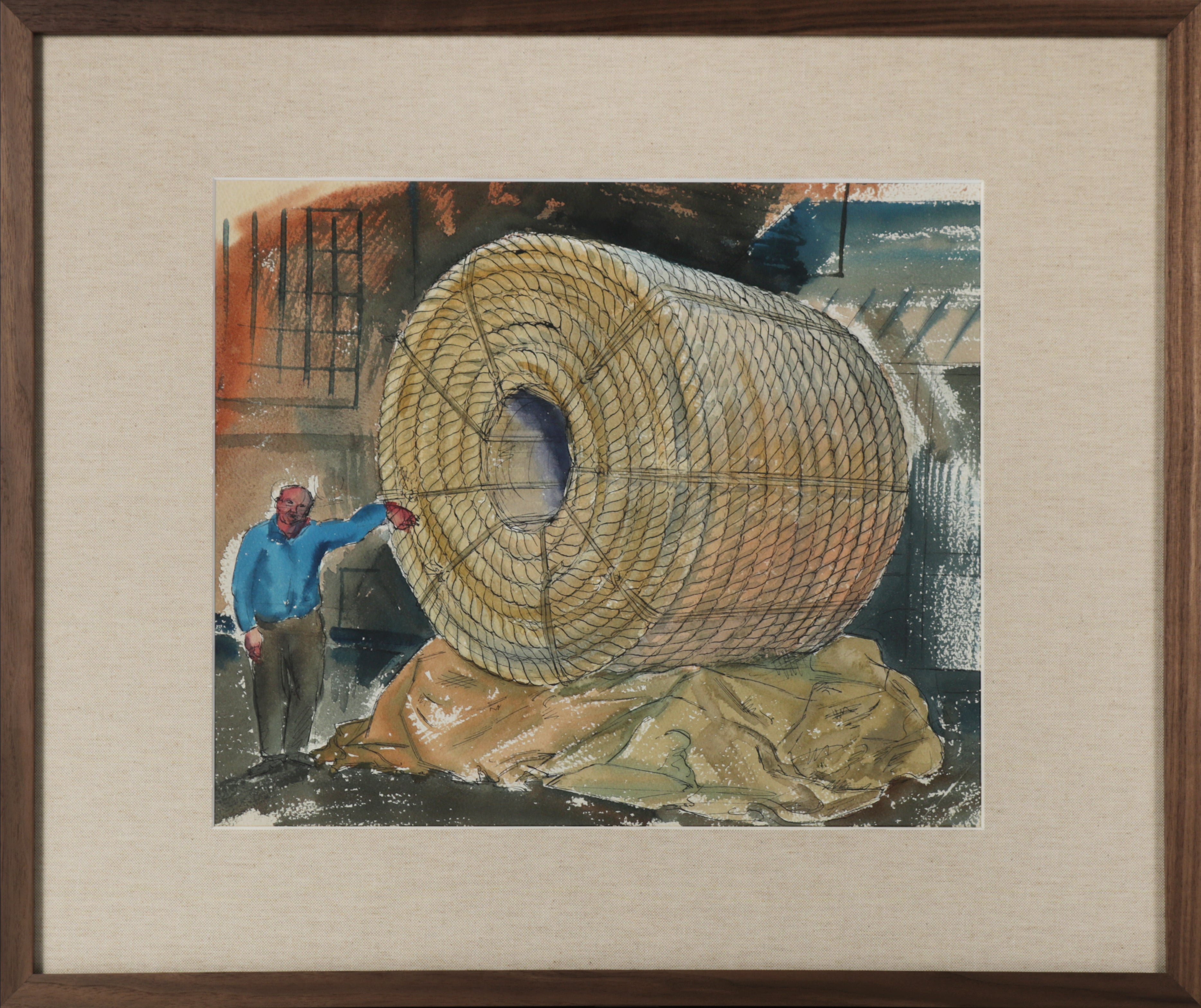This is a photograph of a framed painting, mounted with a textured tan mat and enclosed in a narrow, dark brown wooden frame. The painting, executed in a muted palette of black, gray, orange, yellow, and blue watercolors, depicts a bald Caucasian man in a long-sleeved blue shirt, gray pants, and dark shoes, standing in the lower-left corner of the image. He is positioned on a black floor and appears to be leaning against a colossal cylindrical coil of beige-yellow rope, significantly larger than himself and featuring a hollow center. The massive coil rests on a mound draped with a tan cloth or tarp, suggesting an industrial setting. Behind him, the backdrop hints at the interior of a warehouse or factory.